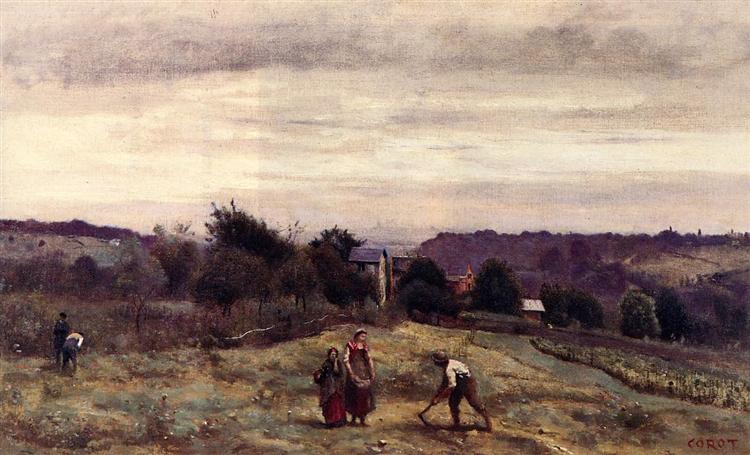This detailed oil painting by Corot features an outdoor scene set in a vast, green field under a dark, gray sky filled with heavy clouds. The setting is enhanced by a backdrop of dark green trees and a couple of indistinct buildings that remain unobtrusive. In the painting, there are at least five clearly visible figures, all dressed in old-fashioned clothing suggestive of a time long past. Two women, donned in long dresses, are centrally situated; one is carrying a basket and appears to be holding up her skirt as if collecting something. Nearby, a man is engaged in farming, wielding a digging implement, possibly a hoe. On the far left, two additional figures are depicted—one of whom is bent over, seemingly picking something from the ground. There is a subtle signature "C-O-R-O-T" at the bottom, identifying the artist and adding a touch of authenticity to this somber yet evocative rural tableau.